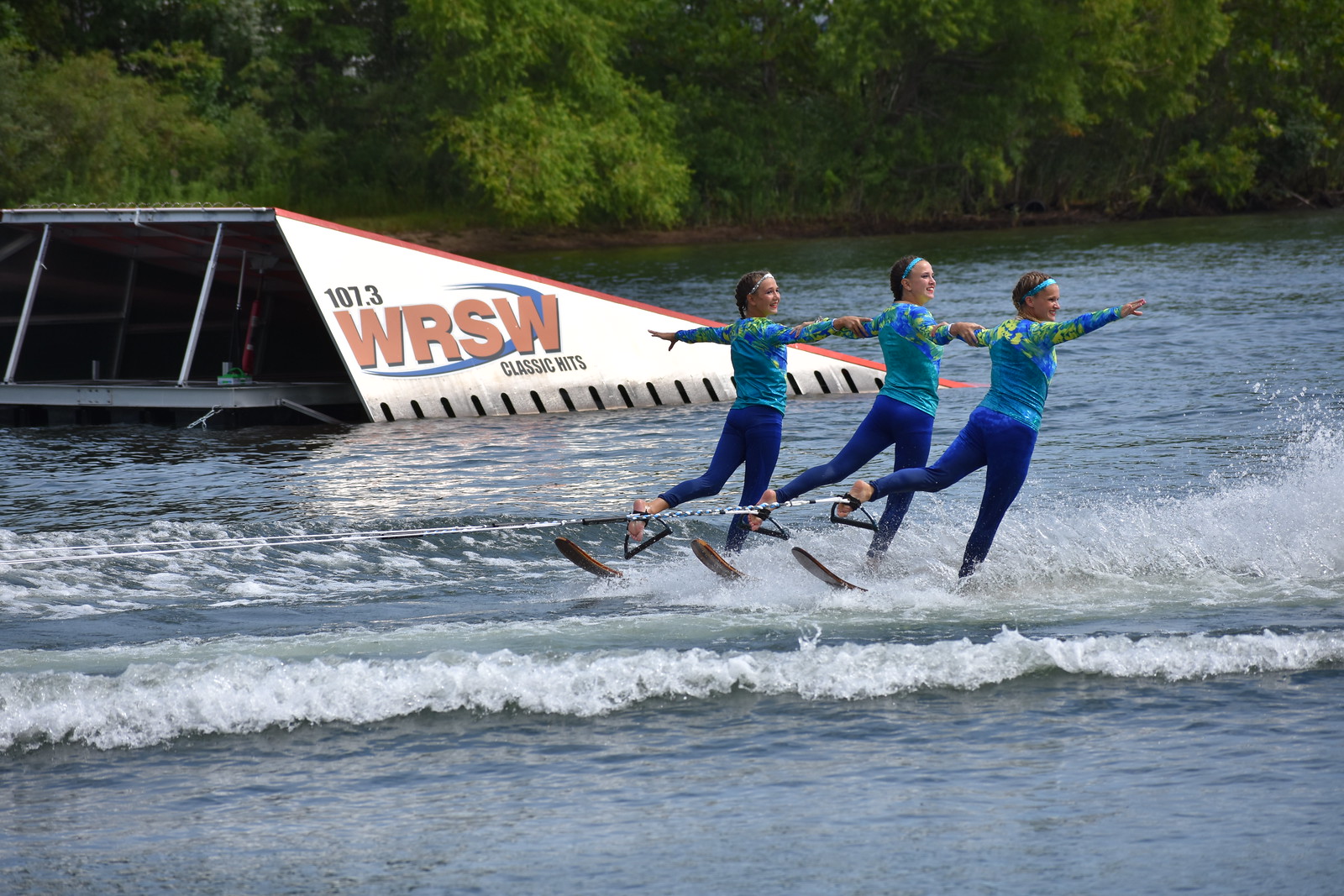In this lively action shot, three young women are captured performing an impressive synchronized wakeboarding routine on a lake. Each woman is outfitted in a matching ensemble of blue and teal full-body wetsuits with yellow-patterned and decorative tops, complemented by teal headbands and their hair neatly braided. They gracefully hold each other's arms, with their free arms elegantly outstretched to the side, and they're balanced on one ski each, with the other leg extended behind them, connected to an unseen boat by a rope. The scene unfolds against the backdrop of the lake's tree-lined shore. In the distance, there is a partially submerged ramp adorned with a sign reading "107.3 WRSW Classic Hits" in yellow letters on a white background, hinting at a promotional event or competition. The white ripples of the wake trail behind the women, adding a dynamic sense of motion to the photograph.